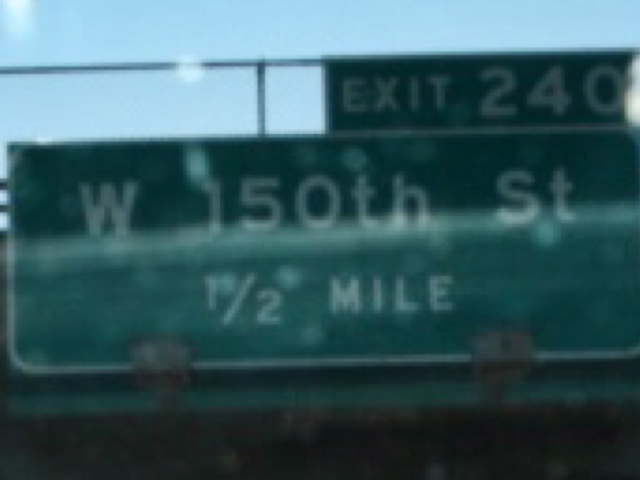The image, taken from a moving vehicle, portrays a slightly zoomed-in and blurry green street sign situated on an overpass or bridge. The upper part of the sign, slightly cropped on the left, reads "EXIT 240" in white, capital letters. Below this, a larger rectangular section displays "W 150TH ST 1/2 MILE". The sky in the background is clear and bright blue, indicating a sunny day. The metal structure holding the sign is partially visible, with sunlight reflecting off the metal components attached to the concrete bridge. The blurriness and pixelation suggest the photo was either taken with some motion or with a significant zoom, providing a sense of depth and perspective to the scene.